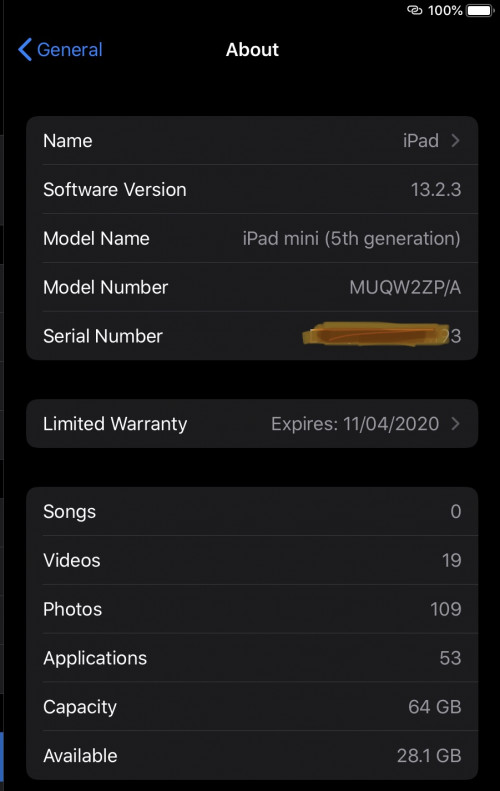The image is predominantly black, with key elements detailed in various sections. In the top right corner, there is a chain link icon indicating 100% battery life. The screen displays several lines of white text against a black background:

- The header includes text stating "The cover lets us name."
- To the right, it says "iPad" with the software version "13.2.3" highlighted.
- Below, the model information reads: "Model Name: iPad mini (5th generation)," "Model Number: MUQW2ZP/A," with the "Serial Number" obscured by a brown bar.
- A section below notes the "Limited Warranty" which expires on "11 September 2020."
- The usage stats are listed: Videos (19), Photos (109), Applications (43), with the capacity at 64GB and 24GB available.
  
A horizontal line spans the screen multiple times, creating separations between different lines of text. The serial number is marked out in brown. The top left corner has a hint of blue, possibly from an icon or status bar. The rest of the image retains a dominant black background, creating a stark contrast with the white text.